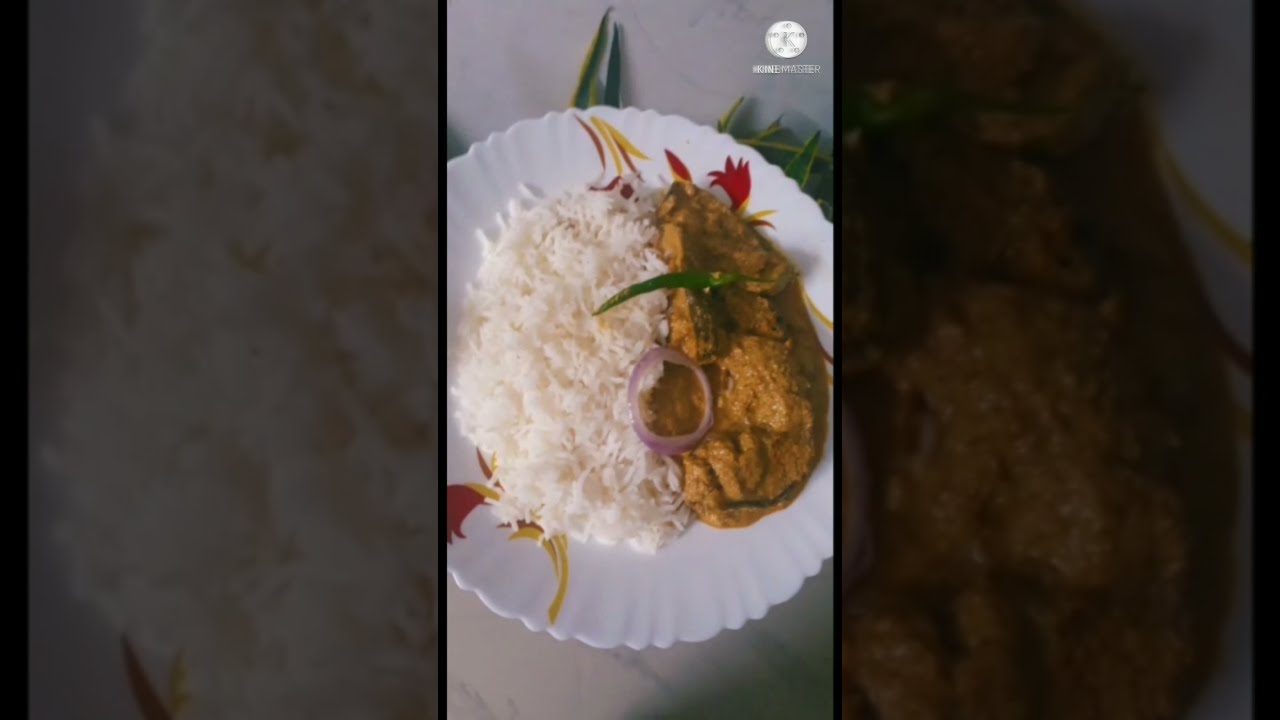This photo captures a culinary dish presented on a round, white ceramic plate with frilly, seashell-like edges. The plate is adorned with a floral print featuring red flowers and yellow leaves and stems. On the plate, the meal is distinctly divided: white rice occupies one side, while the other side holds a brown pureed mixture, possibly resembling an Indian dish like chicken tikka masala. The puree appears to contain chunks of meat, and the dish is garnished with slices of red onion and a green vegetable leaf placed atop both the rice and the puree. The presentation highlights a contrast between the pure white rice and the richly sauced meat, accentuated by the vibrant garnish.